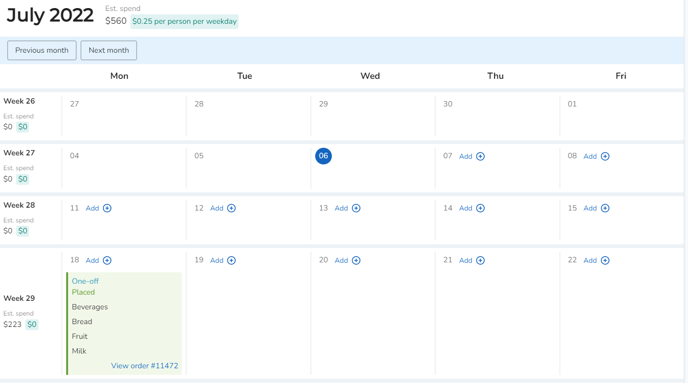This image is a screenshot of a calendar application displayed on a desktop or laptop PC. The interface has a clean design with a white background and light gray dividing lines forming a semi-grid pattern. The grid spaces vary in size; the row being interacted with expands into a large square, while the other rows remain as long, collapsed rectangles.

At the top, the header reads "July 2022" in black text. Below this, it shows the estimated spending amount of "$560" in black text. Additionally, highlighted in green and also written in green text, it states "25 cents per person per weekday."

A blue bar is positioned just below the header, featuring two navigational buttons labeled "Previous Month" and "Next Month." Underneath these buttons, the days of the week—Monday, Tuesday, Wednesday, Thursday, and Friday—are listed out horizontally. Each day forms the top of a respective vertical column. The calendar starts on week 26, with the first day being Monday, June 27th.

A specific row, week 29, is highlighted in green and expanded. It lists various items and notes such as "one-off, placed, beverages, bread, fruit, milk" along with an order number. The established spending for week 29 is indicated as "$223."